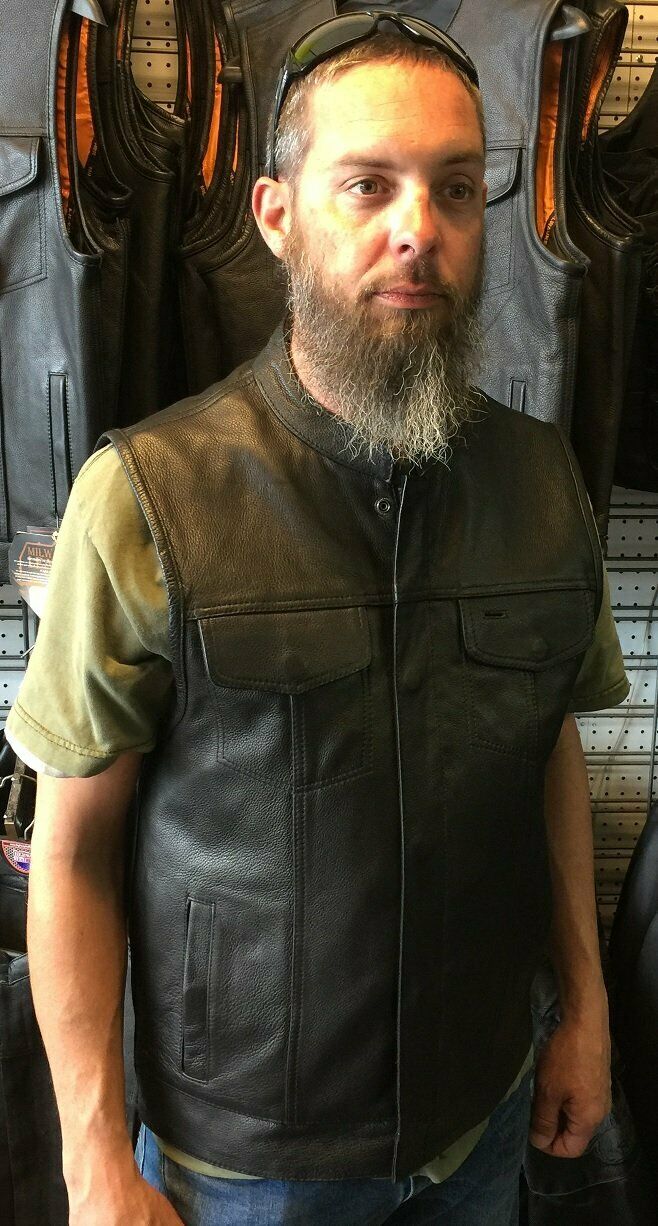In the photograph, a middle-aged man, possibly in his 40s or 50s, stands in a store filled with racks of black leather vests, likely for motorcycle riding. He is modeling a black leather vest with a short collar, which features two chest pockets with button closures and additional hand pockets on the right side. The vest closes via buttons down the center and is lined with an orange, silky-looking material. Underneath the vest, he wears a green t-shirt that peeks out, and he pairs this with blue jeans. The man has very short hair and a long beard that is heavily gray at the tip, matching his graying hair. Perched on top of his head are a pair of black sunglasses. The man is not directly facing the camera but is looking off to his left, raising an eyebrow, and maintaining a neutral expression. The background reveals stacks of leather vests hanging on the wall, which has noticeable holes and gray stripes running horizontally.